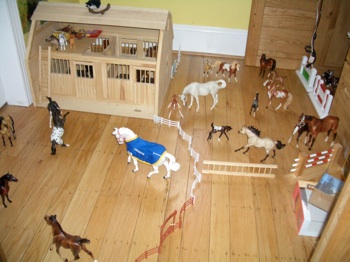The image depicts a highly detailed miniature livestock barn setting within a house, meticulously designed to resemble an aerial view of a stable and horse ranch. This intricate play scene features various fenced-in areas separated by distinct red and white barriers. 

In the top left corner, a barn with four stalls houses several horses. Adjacent to this, on the top right, is a penned section filled with horses of varying ages, from colts to full-grown adults, including one horse adorned with a blue blanket. The scene is animated with the presence of a person dressed in a black shirt, white pants, and riding boots, walking or running among the horses. 

Another notable section on the bottom right is an empty, fenced-in area without any animals. The carefully arranged layout, with detailed representations of fences and the person interacting with the animals, makes the miniature setting strikingly realistic, as if viewed from a helicopter above an actual ranch.